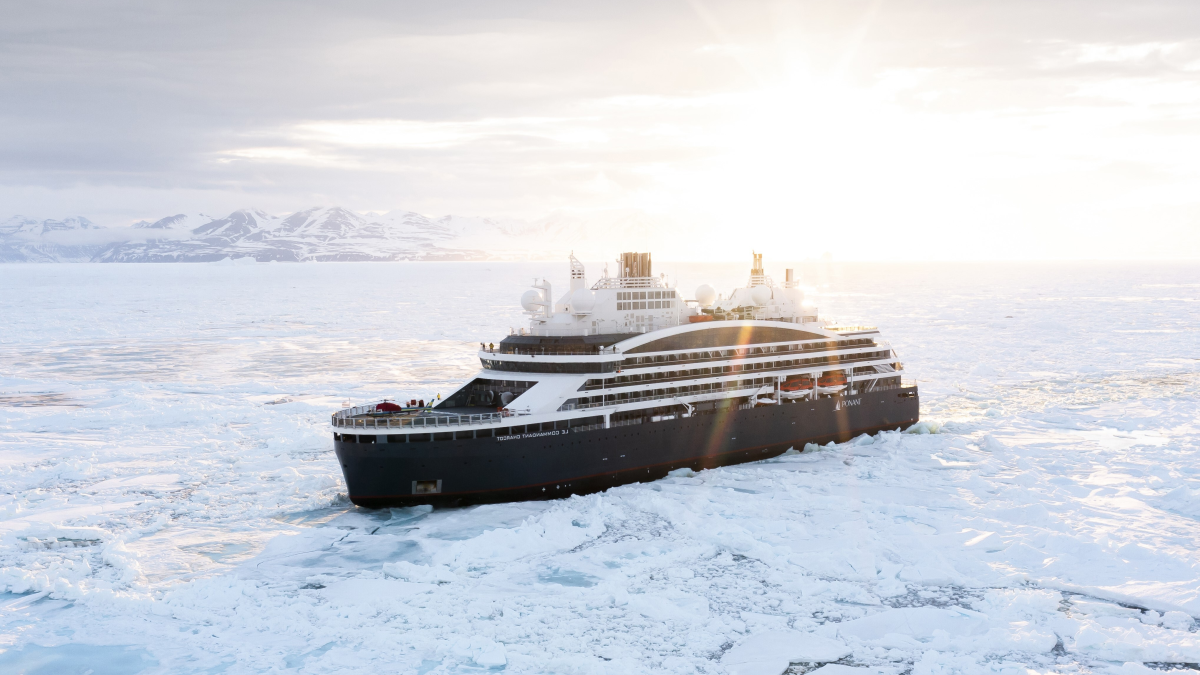In a breathtaking photograph taken outdoors, a large cruise ship is navigating through the icy waters of the Arctic or a similar polar region, possibly even Antarctica. The ship’s dark gray lower body is complemented by white trim and housing units on its many levels, with a striking red line at the bottom. On deck, lifeboats and various white structures, including spherical elements and steam towers, are visible. Surrounding the ship, the ocean is nearly entirely covered in patches and chunks of ice, which the ship appears to be breaking through, leaving a trail of open water behind it. To the far left, a snow-covered mountain range is visible under a canopy of white and gray clouds. Further off in the distance, the sun breaks through, casting a bright, yellowish glow over the scene and illuminating the otherwise cloud-filled sky. The area is clearly frigid, with the vast landscape dominated by snow and ice. The overall scene is one of stark natural beauty and human engineering, blending harmoniously under the bright, Arctic sky.